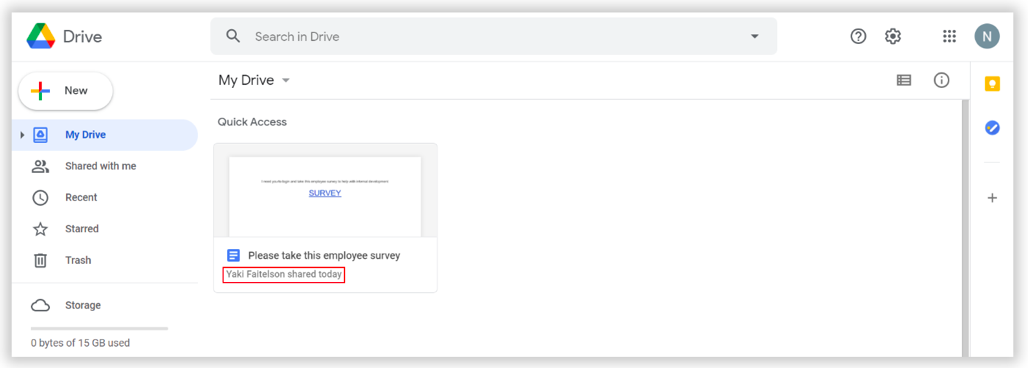Detailed Caption: 

This image showcases the Google Drive interface. Prominently displayed in the top left corner is the Google Drive logo, accompanied by the text "Drive". Directly adjacent to this is a search bar with the placeholder text "Search in Drive". To the right of the search bar, several icons are visible: a question mark for help, a settings gear for configuration options, a menu icon, and a circular user profile indicator featuring the letter 'N', likely representing the user's initial.

On the left-hand side of the interface, there's a vertical navigation bar with various options. At the top is a button to add a new file. Below this, a series of category options are listed, each with a corresponding icon: "My Drive" (highlighted in blue, with a computer icon), "Shared with me" (two silhouettes), "Recent" (a clock), "Starred" (a star), "Trash" (a trash can), and "Storage" (a cloud). 

At the bottom of the sidebar, storage information reads "0 bytes of 16 GB used". Because "My Drive" is selected, the main portion of the screen displays its contents under the heading "Quick Access". A red box highlights a survey titled "Please take this employee survey," shared by Yaki Fulteson on the current day.